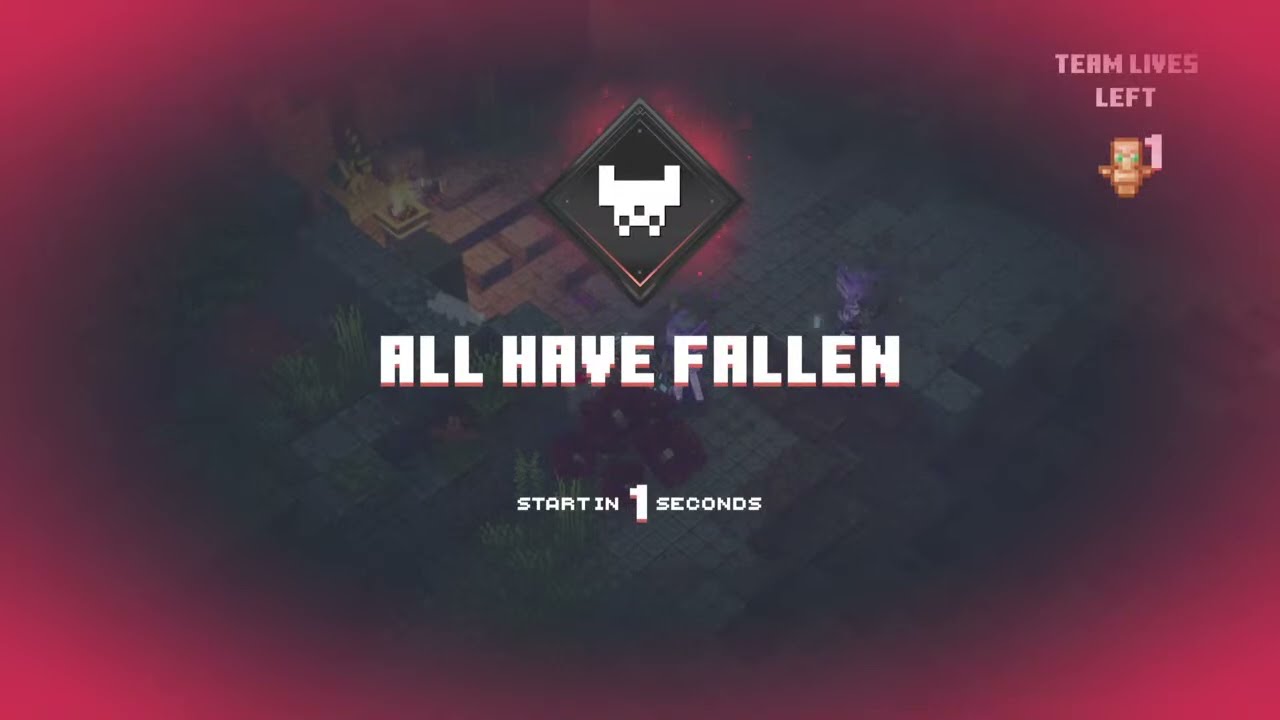The image depicts a paused moment from a mobile or tablet video game, surrounded by a smoky, gradient border that transitions from a pronounced rosy pink in the corners to a darker, hazy purple around the edges, ultimately blending into a grayish-black towards the center. Centralized within the image is a pixelated, all-uppercase white text that reads "ALL HAVE FALLEN," with a black diamond-shaped logo overlapping the letter "E," showing a simplistic sprite character. Below this text, the message "Start in one second" indicates an imminent restart. In the upper right corner, the text "Team Lives Left: One" is displayed next to a small, brownish creature or golden robot holding a numeral one. The background seems to depict a 3D, third-person platform game environment, featuring elements like flowers, bushes, grasses, a stone walkway, and a small area with smoke, suggestive of a burning spot, partially obscured by the pink hue.